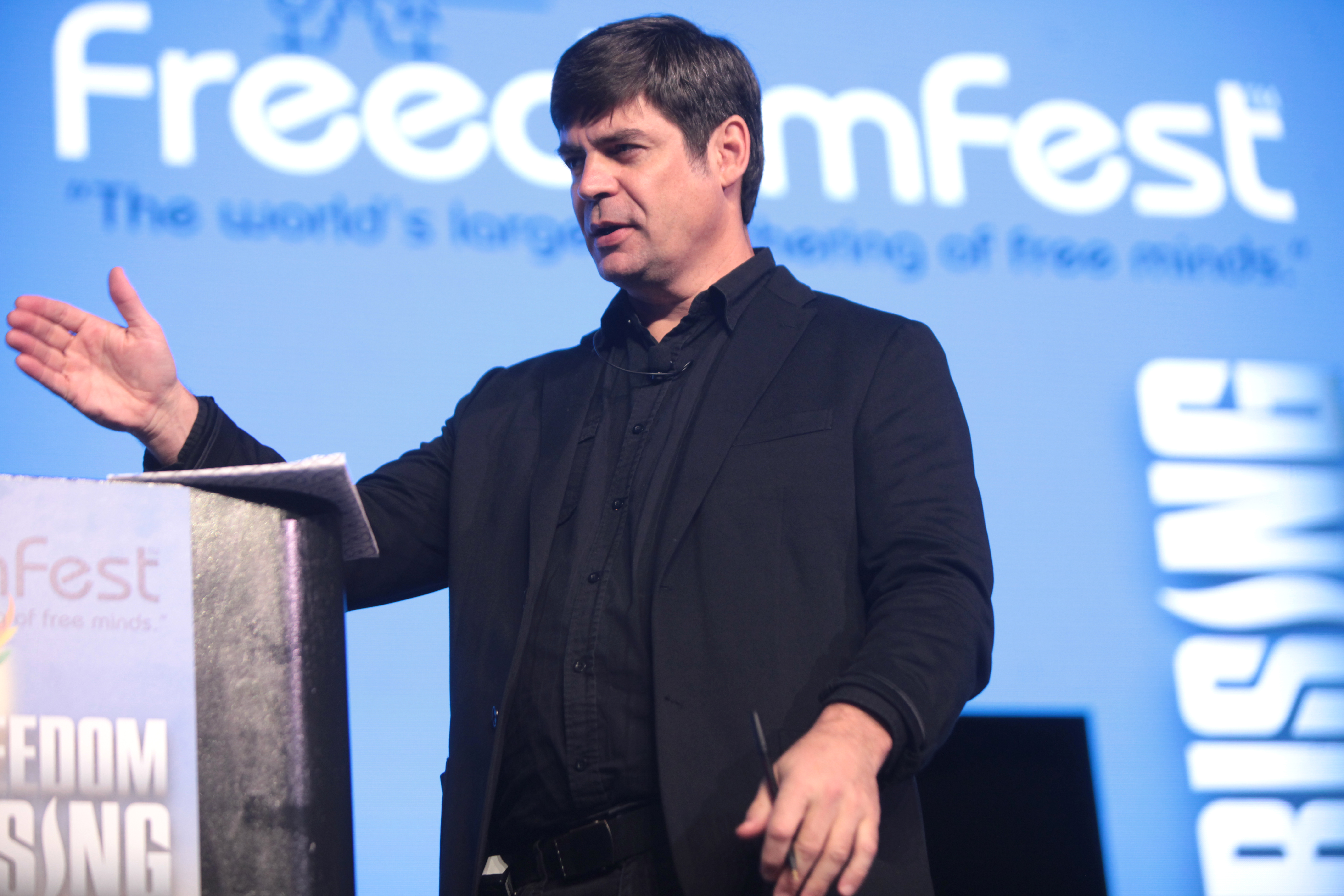This image captures Nick Gillespie, a white male presumed to be in the age range of 45 to 50, standing on a stage at Freedom Fest. He has medium-length black hair showing hints of gray and is dressed entirely in black, including a button-up undershirt, a jacket, pants, and a belt. He has a black microphone clipped to his shirt and is gesturing with his right hand, which holds a black pen. He stands beside a black podium that has a stack of papers or notebook on top of it. The podium is also emblazoned with the words "Freedom Fest," while the blue background banner behind him reads, "Freedom Fest, the world's largest gathering of free minds." The visual context suggests he is delivering a speech at this event, addressing an audience.